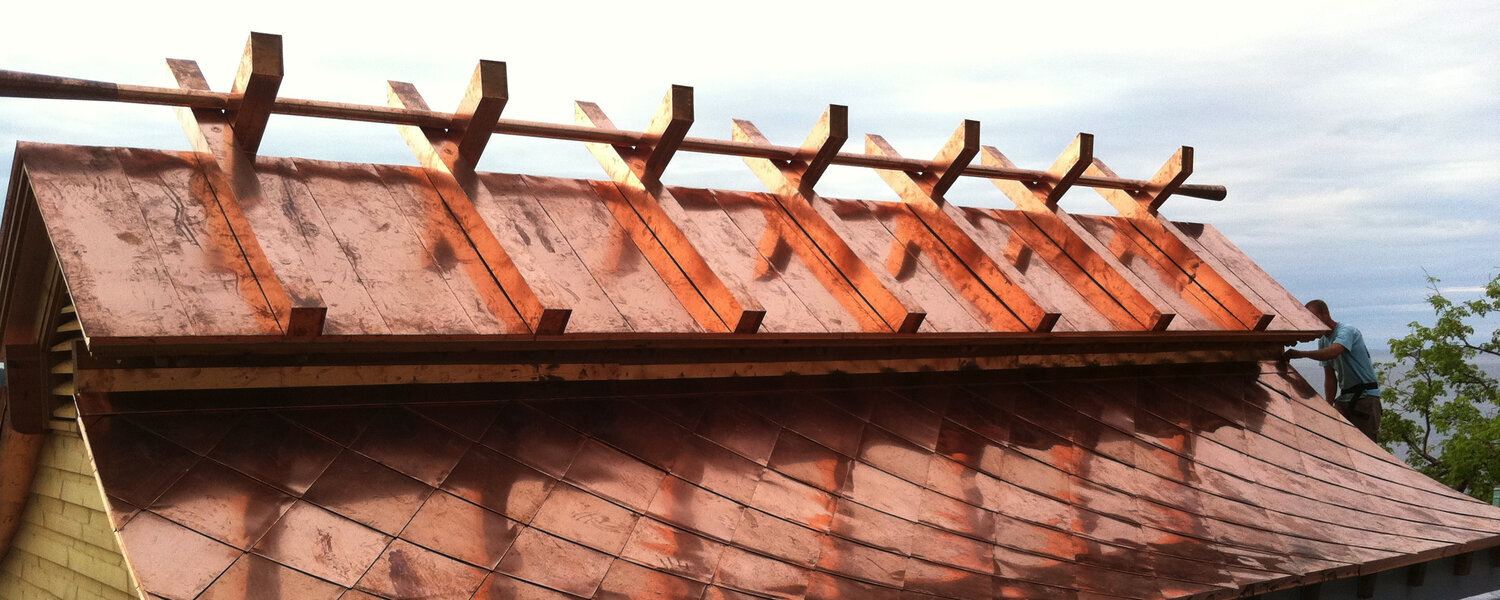This is a detailed photograph of the peaked roof of a building, styled in a Viking theme. The roof is predominantly clad in shiny copper-colored squares which give it a reflective quality. The roof consists of two primary layers, with a copper-colored slant about two feet long. The pinnacle of the roof features a unique structure composed of six or seven Y-shaped beams, possibly more, that ascend towards the sky. A wooden rod rests horizontally atop these beams. The apex also includes a roof vent. The building facade beneath the roof is clad in yellow wood with trim separating the different roof sections, complemented by a section that is reminiscent of snakeskin in texture and is also a shiny red color. In the background, there's a builder dressed in a blue shirt and khaki shorts, working on a ladder, with green trees and a blue sky visible behind. This combination of elements makes for an aesthetically striking roof design.